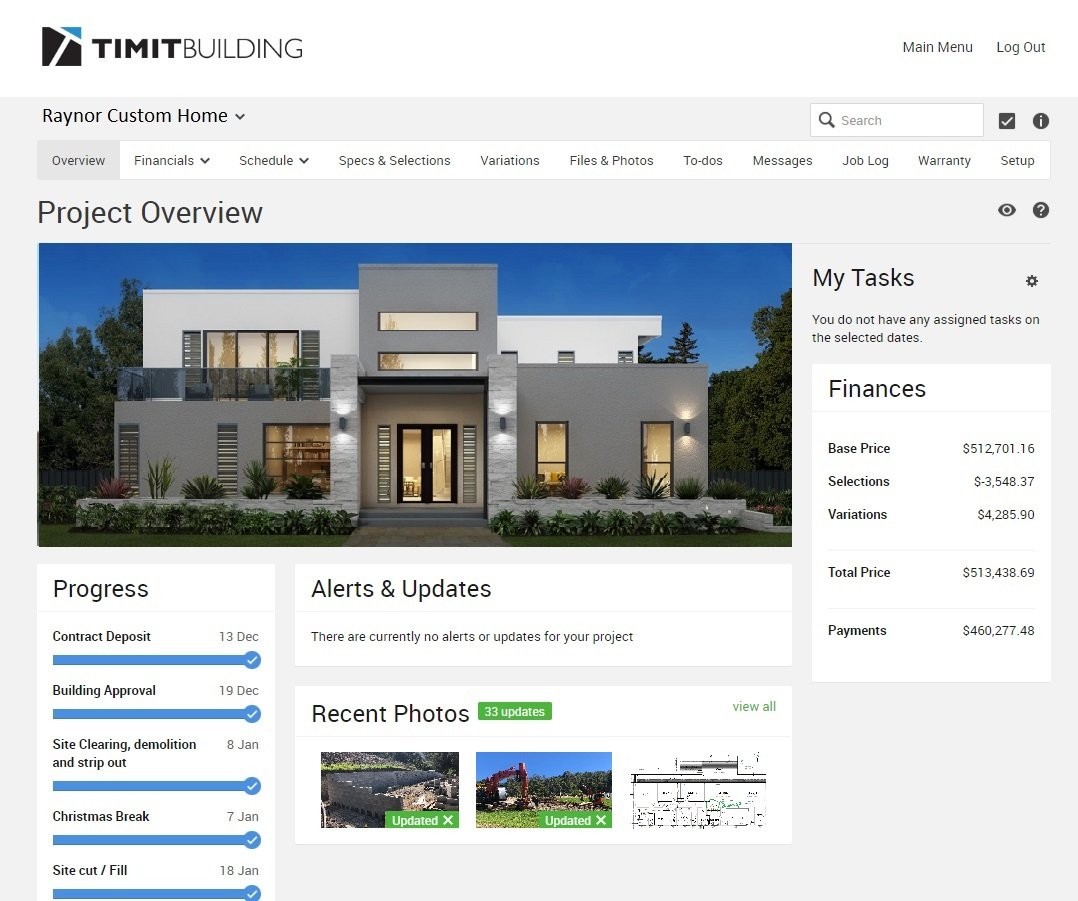This screen capture showcases the webpage for the TIMIT Building project, specifically under the Raynor Custom Home section. The top of the page features a detailed menu bar with tabs labeled: Overview, Financial, Schedule, Specs, Selections, Variants (or possibly a similar term, though it's not clear due to an unusual font), Files and Photos, To-Dos, Messages, Job Log, Warranty, and Setup. The currently selected tab is Project Overview.

The central part of the screen displays the front view of a modern, flat-roofed house under the label "Progress," indicating that all listed construction steps have been approved. Below, recent photos of the job site provide visual updates on the house's development. The purchase price for this custom-built home is prominently displayed as $513,438.60.